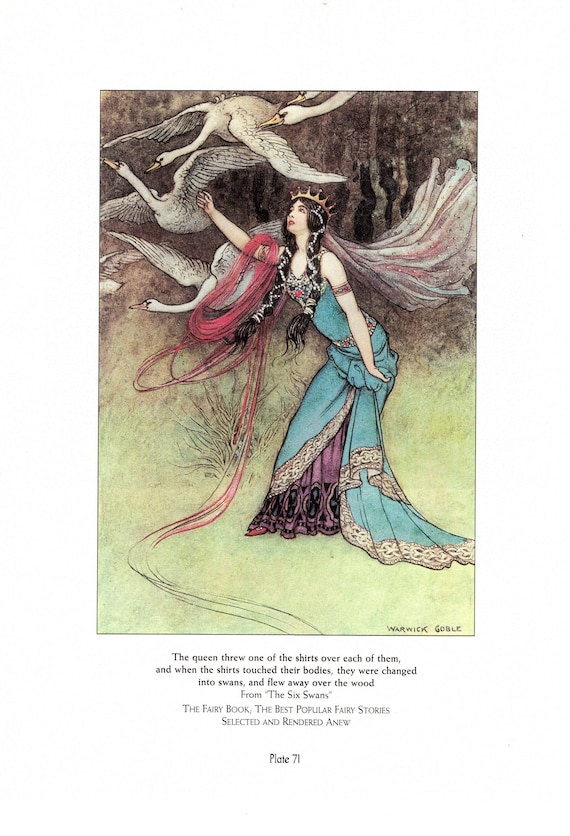The image is a watercolor-style illustration depicting a queen with long black braided hair, adorned with a crown, wearing an intricately designed dress. Her royal gown is green with golden borders and features maroon and purple designs at the bottom. She stands in a green field, raising one hand as if casting a spell. Around her shoulders, she has silver ornaments, and a trailing red yarn is wrapped around her arm. Above her, swans are flying into the air, symbolizing transformation. In the background, there are hints of trees or mountains. The illustration includes text at the bottom in black: "The queen threw one of the shirts over each of them, and when the shirts touched their bodies, they were changed into swans and flew over the wood." Further down, it reads, "from The Six Swans, The Fairy Book, the best popular fairy stories, selected and rendered anew," followed by "Plate 71" in bold text. At the bottom right, the artist's name, Warwick Goble, is signed.